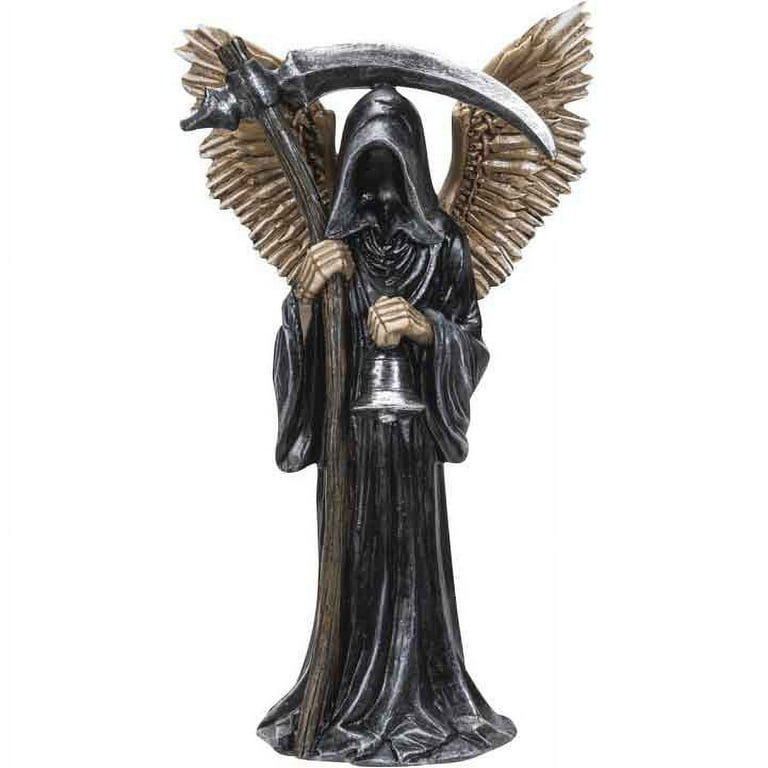The image depicts a highly detailed, metallic sculpture of the Grim Reaper adorned with gold wings. The figure is shrouded in a black, hooded robe that completely obscures its face, with long, flowing sleeves draping down. The hood and robe create a ghostly silhouette as they sweep to the ground, forming the base of the statue. In its left hand, the Grim Reaper holds a silver bell that hangs ominously, while in its right hand, it brandishes a massive sickle with a wooden pole and a gleaming blade extending above its head. The gold wings, extending from its back, strikingly contrast with the predominantly black and gray figure. The meticulous highlights on the robe give the sculpture a polished, metallic appearance, enhancing its eerie, lifelike quality. This piece seems to be a professional product image, likely intended for sale on a website, given the lack of background.